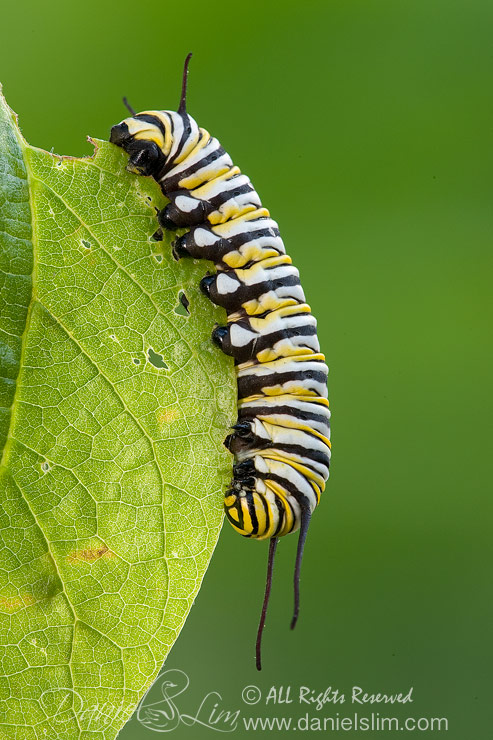This is a highly detailed, close-up photograph of a large, fat caterpillar with a striking pattern of black, white, and yellow stripes along its body. The caterpillar is positioned on the edge of a green leaf, appearing to have eaten parts of it, as there are noticeable holes and damage on the leaf. The caterpillar has black legs with white dots, and distinctive antenna-like appendages at both its head and tail, likely serving as a defense mechanism against predators. The leaf, shown from the backside, reveals intricate details such as its fractal-like patterns and internal structures, enhanced by the well-focused shot. The background is a blurred green, which contrasts with the sharp, vibrant details of the caterpillar and leaf. In the lower right corner of the photo, there is white text that includes a signature, the URL danielslim.com, and a copyright notice stating "all rights reserved."